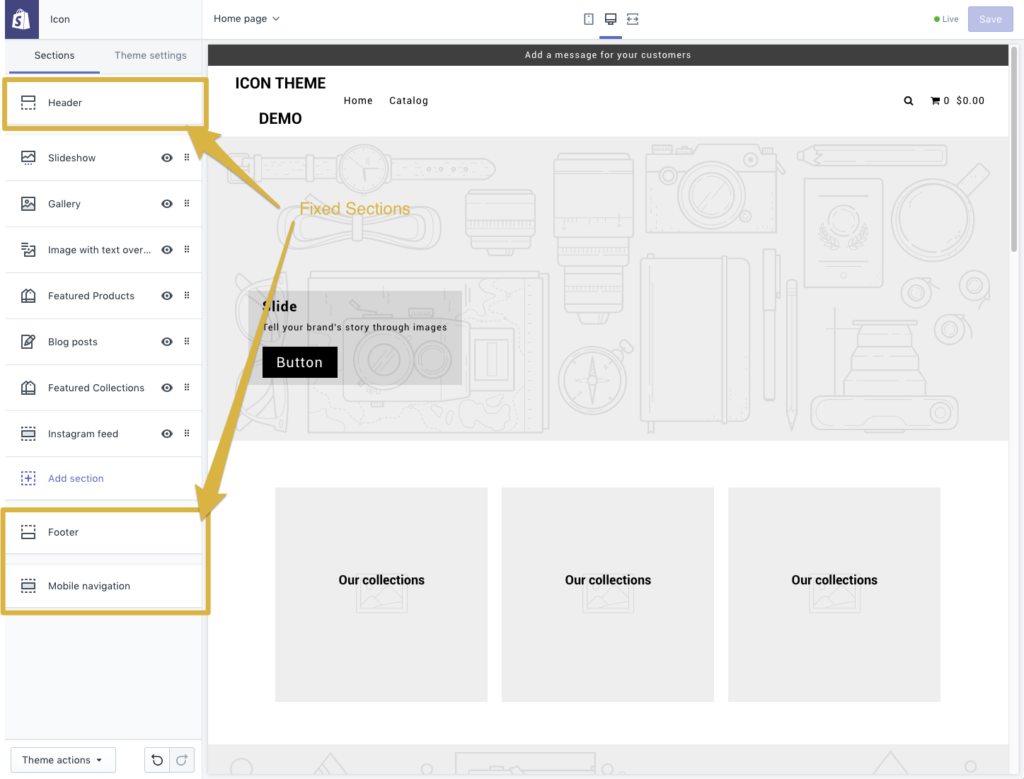The white-background webpage screenshot showcases a detailed and organized layout, designed with a shopping theme in mind. 

On the left side, at the top, an orange square contains a slightly angled, purple shopping bag icon featuring an 'S.' Below it, the sections panel presents various navigational options in smaller black font, including "Sections" and "Theme Settings." The top item in this panel, labeled "Header," is highlighted in an almost golden shade, accompanied by a similarly colored arrow pointing to its bottom right corner. Other items listed include "Slideshow," "Gallery," and "Image with Text Over," each with corresponding symbols. Additional features such as "Featured Products," "Blog Posts," "Featured Collections," and "Instagram Feed" are indicated by dashed-line boxes with plus signs inside them. Within this boxed area, the words "Fixed Sections" appear at the top, guiding a long arrow that points downward to "Footer" and "Mobile Navigation" at the bottom.

In the middle section of the webpage, a slender black banner spans the top, displaying the message "Add a Message to Your Customers" in white font. On the top left corner of this section, the text "Icon Theme" appears in larger black font, with the word "Demo" directly below it. The middle part of the header includes navigation links "Home" and "Catalog" in smaller black font. 

The central feature of the webpage is a large, faded blue box containing various neatly arranged items, reminiscent of objects laid out on a table: a passport, watch, compass, camera, magnifying glass, pencil, couple of pens, and a smartphone.

At the very bottom of the page, three similarly styled faded baby blue boxes are evenly spaced. Each box is labeled "Our Collections" in black font, providing clear sections for featured content.

This structured and visually appealing webpage layout reflects the meticulous work of a graphic designer, focusing on a theme suited for showcasing products and facilitating user navigation.